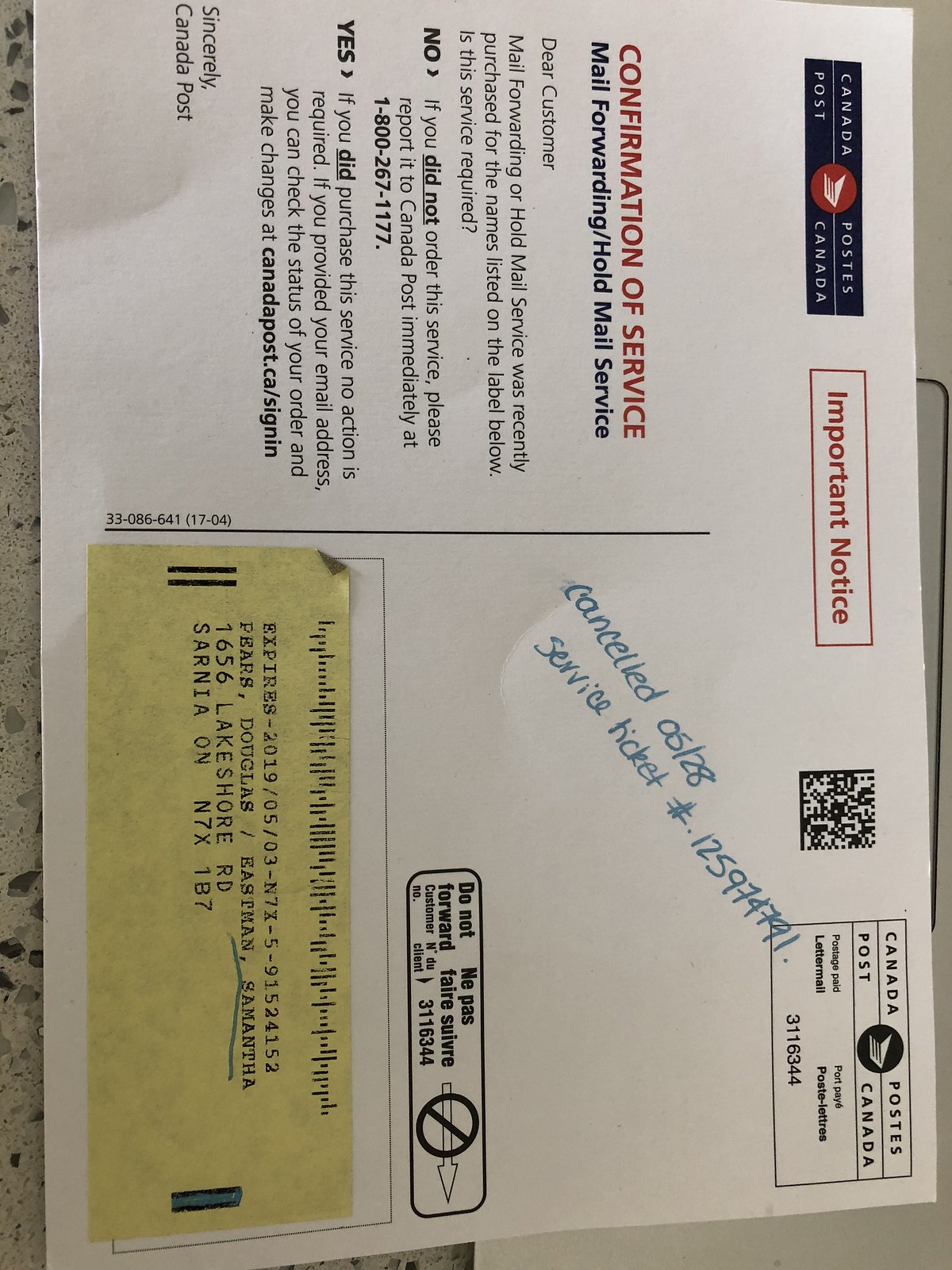The image depicts a piece of mail from Canada Post oriented 90 degrees clockwise. At the top of the mail, there is a vertical line dividing it into two halves. On the left side, the heading reads “Important Notice” above the text: “Confirmation of Service, Mail Forwarding, Hold Mail Service.” Below that, the letter addresses the customer, stating, “Dear Customer, Mail forwarding or hold mail service was recently purchased for the names listed on the label below. If this service was not required, please report it to Canada Post. If you did purchase this service, no action is required.” The letter is signed off with “Sincerely, Canada Post.”

On the right side of the mail, the Canada Post logo is at the top right, and a blue handwritten note reads “Canceled 0528 Service Ticket” along with the service ticket number. At the bottom of the right side, there is a yellow sticky note on the area meant for the address. The sticky note contains the new address where the mail is supposed to be forwarded. The overall color scheme includes white, yellow, and various shades of blue. The mail piece, with details such as the “Canceled” note and additional instructions about reporting or confirming the service, appears to rest on a desk.